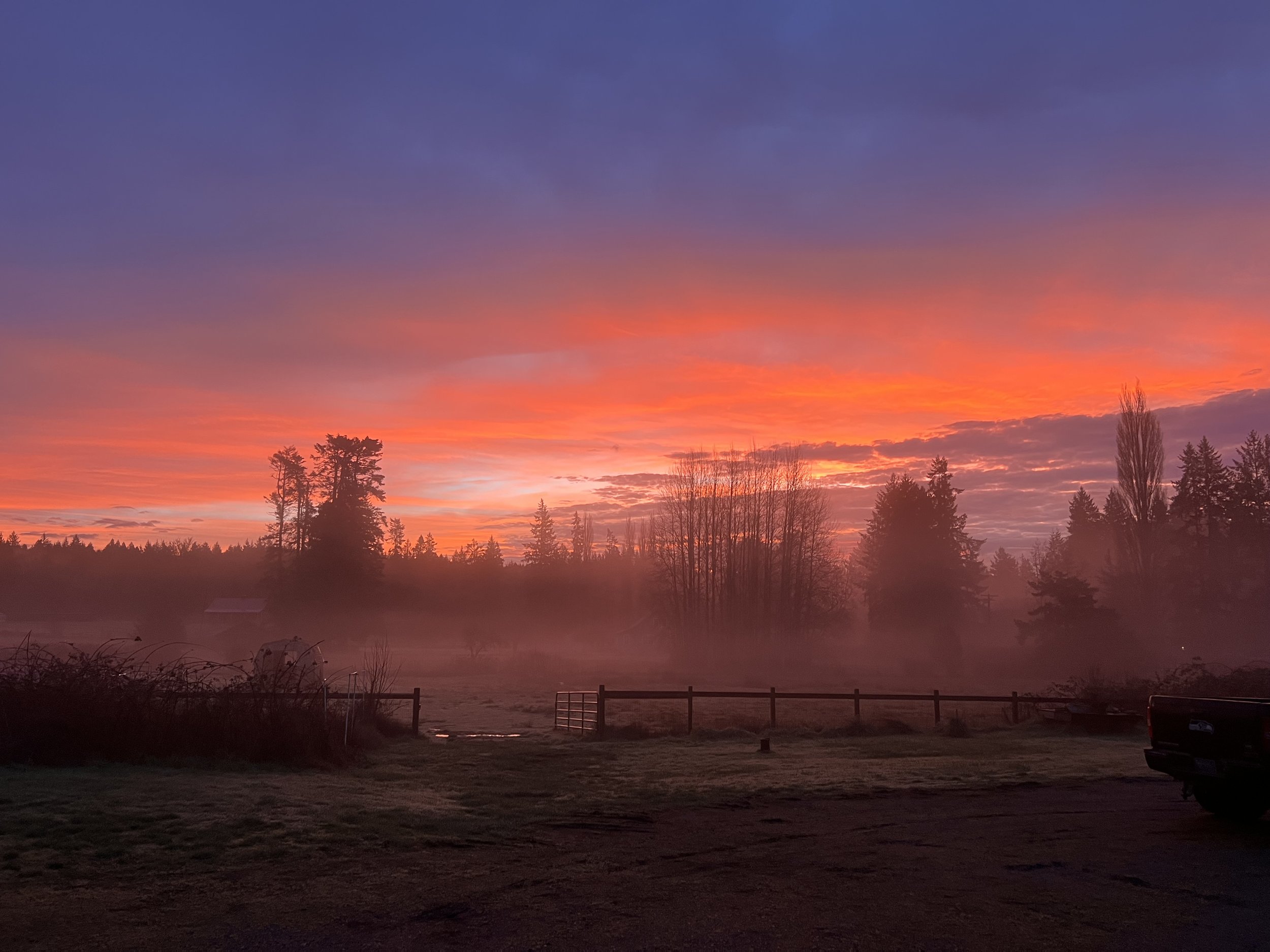The image depicts a tranquil scene, either at sunrise or sunset, set in a large, mostly flat field. In the foreground, patches of dirt and grass are visible, illuminated by the warm, glowing hues of orangish, reddish, and pinkish colors from the sun low on the horizon. The sky overhead transitions to deep shades of blue and purple, with pockets of bluish and purple clouds, particularly on the right.

A wooden fence spans horizontally across the middle of the photograph, featuring an open gate that allows a glimpse into the background. Just behind this fence, there's a pervasive thick fog or mist that obscures some of the details but adds a mystical quality to the scene. Silhouettes of numerous trees line up behind the mist, creating a layered effect, with some trees appearing barren, especially the one at the center.

On the lower left side of the image, partially hidden by the fog, stands a farmhouse next to a large tree. Further to the lower right, the back of a pickup truck is barely discernible, parked on what looks like a dirt road bordered by grass in the foreground. This dirt road leads up to the fenced-in area, complementing the rustic atmosphere of the scene.